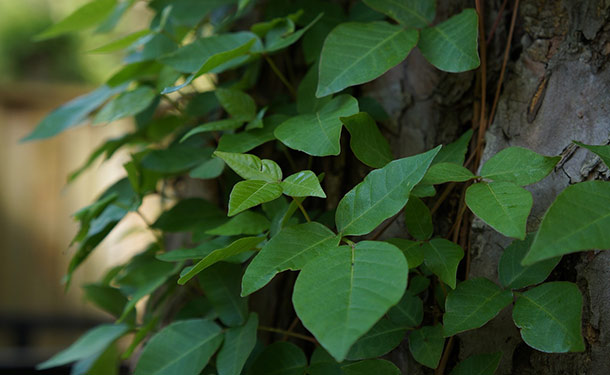This close-up image features a cluster of vibrantly green leaves, each characterized by a pointed shape and arranged in groups of three. The leaves exhibit a gradient of green hues, with the smaller, younger leaves appearing lighter and the older, mature ones darker. The foliage is seen climbing a surface that could potentially be tree bark or a stone wall, identifiable by its grayish-brown texture. The primary cluster, prominently displayed in the front center-right of the image, is sharply focused, showcasing the leaves' detailed structure. Towards the left, the leaves progressively blur into the background, which is composed of a mix of greens, tans, and browns, ultimately fading into an indistinct, blurred backdrop. Additionally, two golden-brown vines intertwine with the leaves and the textured surface, enhancing the natural theme of the image. The background also includes a very blurred brown fence, suggesting the foliage is at the base of a tree or climbing up a structure in a natural setting.